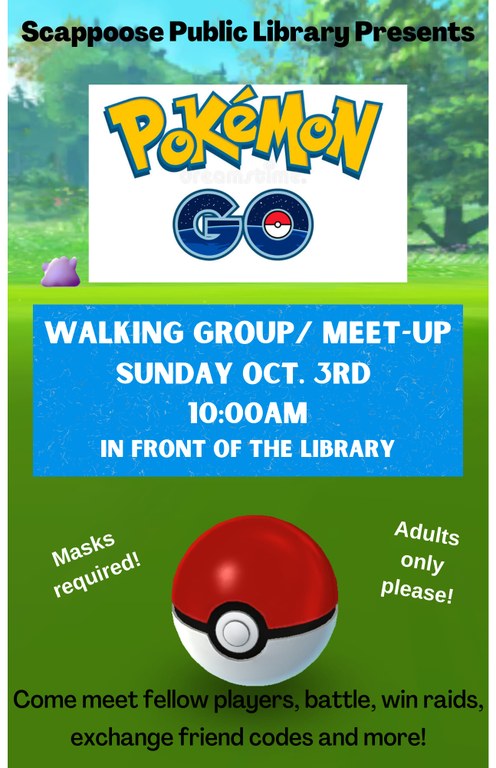The image features a vertical advertisement for a Pokémon GO event hosted by Shnappoo's Public Library. At the top, black text reads "Shnappoo's Public Library Presents." Directly below, a white box prominently displays the iconic Pokémon logo. The logo features "Pokémon" in bright yellow letters outlined with a muted blue, and beneath it, "GO" appears in dark blue with a starry effect. The "O" in "GO" contains a Pokéball, which has a red upper half, a white lower half, and a central black circle divided by a line.

The middle section showcases a blue rectangular box with white text announcing the event details: "Walking Group/Meetup, Sunday, October 3rd, 10 a.m., in front of the library." The background of the advertisement is a green, outdoor Pokémon setting, complete with a tree in the upper right corner.

Below the event details, another image of a more detailed Pokéball is featured, reflecting light from its surface. Flanking the Pokéball, the text reads "Masks Required" on the left and "Adults Only, please" on the right, both in white. At the bottom of the advertisement, black text outlines the activities: "Come Meet Fellow Players, Battle, Win Raids, Exchange Friend Codes, and more."